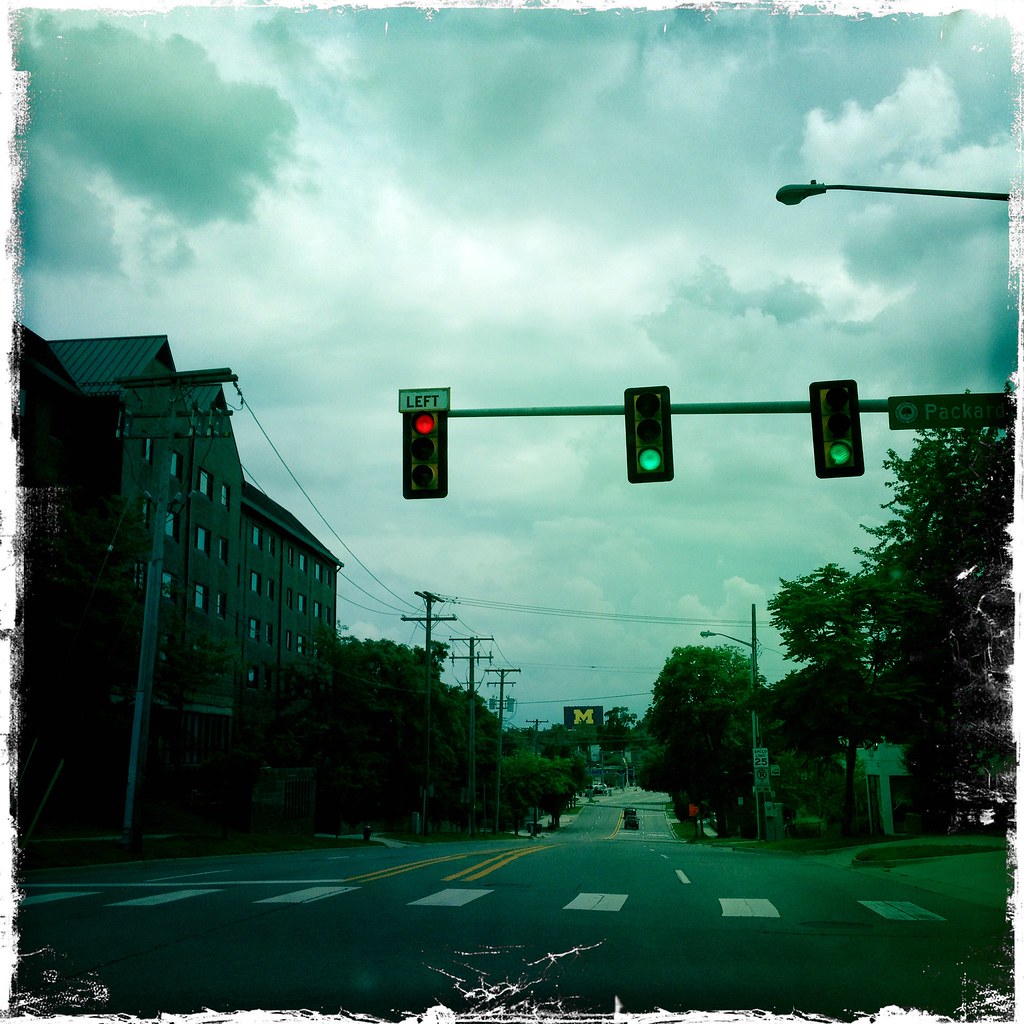This evocative nighttime street scene captures a moody urban atmosphere with a rich array of details. The photograph, framed in a square but with uneven, scraped, and scratched edges, reveals a cloudy sky painted in various shades of gray and white. The perspective is set from the vantage point of a crosswalk, whose distinct white stripes are prominently visible at the bottom of the image. Extending into the distance is a long road marked by a double yellow centerline, flanked on either side by dashed white lane indicators.

In the far background, a luminous sign displaying the letter "M" in yellow adds a splash of color to the scene, hinting at a popular or significant location. Closer to the viewer, three traffic lights punctuate the twilight; the nearest light shines red, the middle one glows green, and the last also glows green but features a black and white "left" arrow affixed to the red symbol. To the left side of the street, buildings line the road, subtly framing the scene and adding to the sense of an urban landscape bathed in the stillness of night. The distant cars add a touch of life to the otherwise tranquil environment, completing this atmospheric visual narrative.